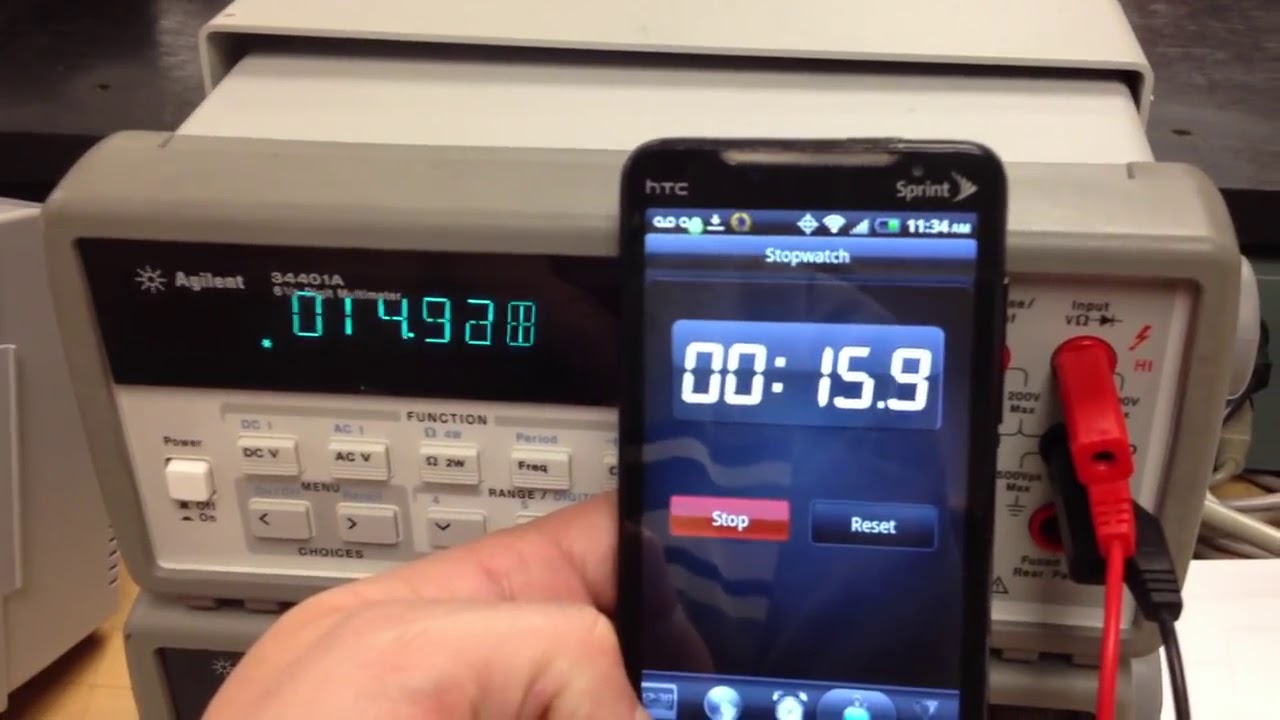In the image, a person's hand is visible holding a Sprint HTC smartphone slightly to the right of the frame. The phone's screen displays a stopwatch timer reading 15.9 seconds, along with the stop and reset buttons. Behind the phone, there is a digital multimeter with the model number Agilent 34401A. The multimeter features a digital readout displaying the number 14.928 and a variety of functions including DCV, ACV, frequency, power off, power on, and various input options. Red and black connections are inserted into the input sockets of the multimeter. The multimeter itself is primarily white with grey trimmings. The scene suggests the person is using the phone's stopwatch function while simultaneously working with the multimeter.